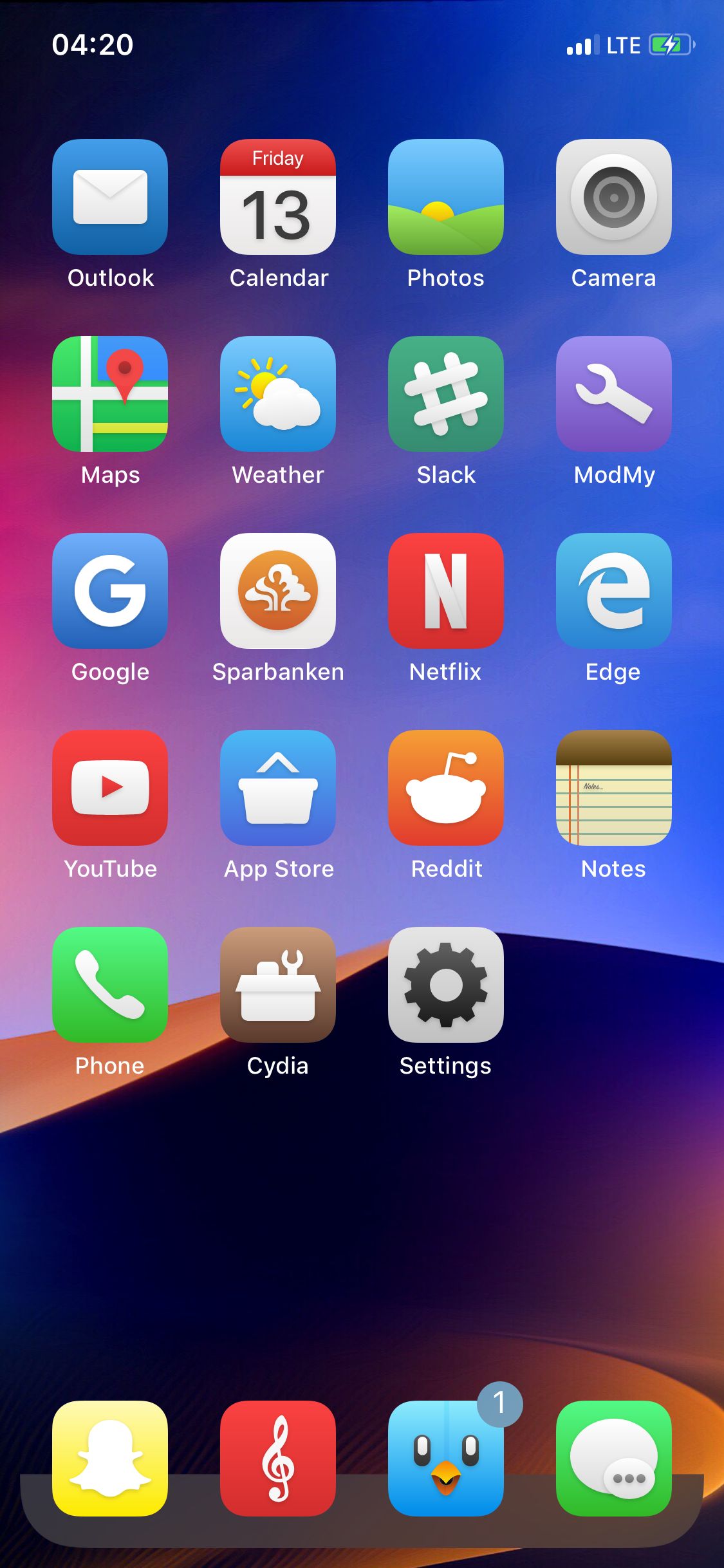The cell phone screen displays a status bar at the top with the time "4:20" on the left, and icons for cellular signal strength, LTE connectivity, and a battery indicator showing that the device is being charged. Below this bar are four rows of app icons. The first three rows each contain five icons, while the fourth row contains four icons. From top to bottom, left to right, the apps displayed are: Outlook, Calendar, Photos, Camera, Maps, Weather, Slack, ModMy, Google, SparBanken, Netflix, Edge, YouTube, App Store, Reddit, Notes, Phone, Cydia (C-Y-D-I-A), and Settings.

At the very bottom, there are four notable icons: a yellow alarm clock, a red music app, a blue Twitter app with a notification badge displaying the number one, and a green messaging app. The background wallpaper features a serene landscape of sand dunes beneath a clear blue sky.

The array of icons includes a vibrant mix of colors: red, blue, green, yellow, orange, brown, pink, purple, white, black, gray, and various shades of brown and green. The overall screen is a colorful and organized display of the user's most-utilized applications.